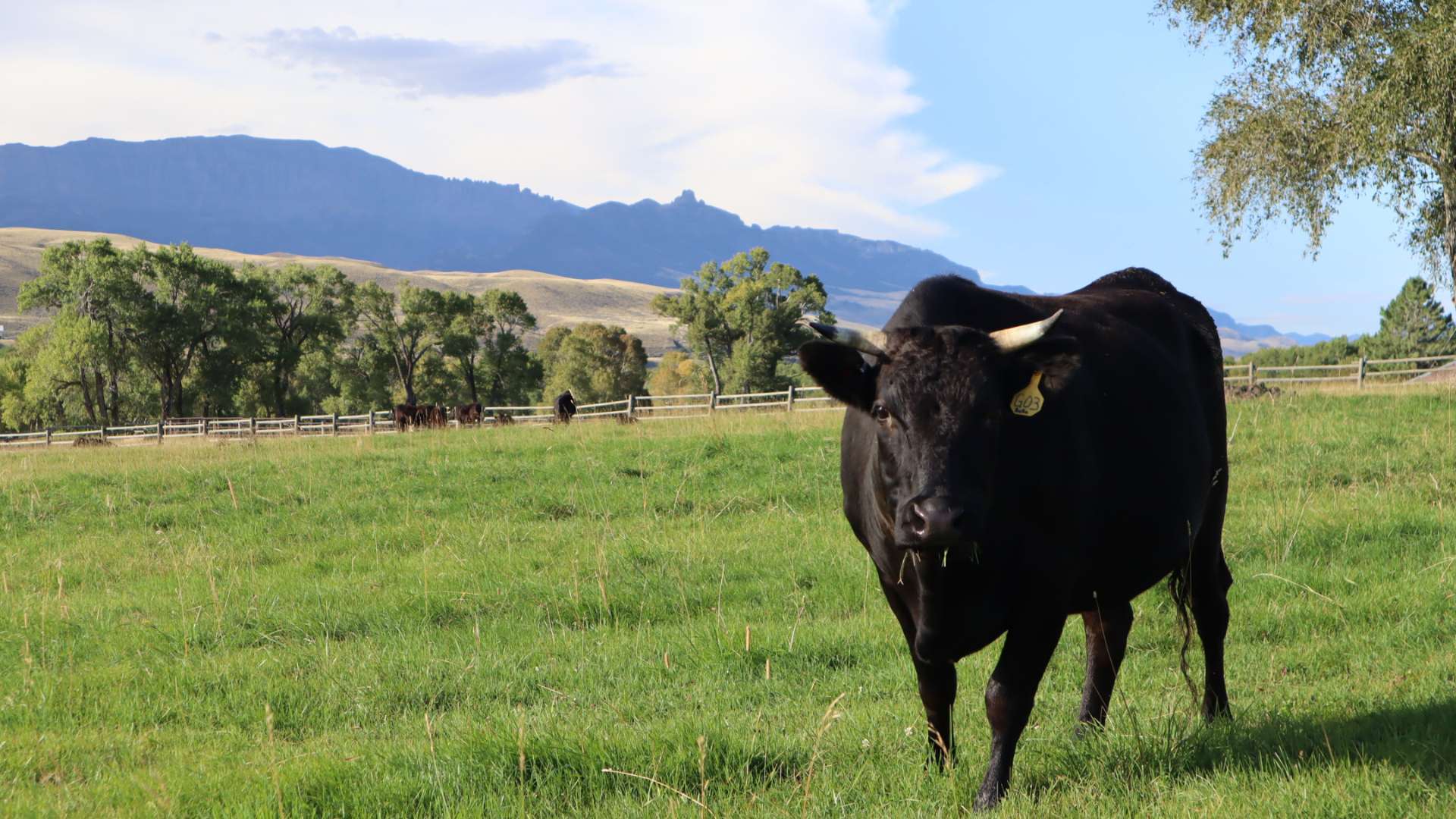The image captures a picturesque countryside scene, prominently featuring a solitary bull in the foreground on the right-hand side. The bull, strikingly all-black, stands in a lush, grassy field dotted with clover and wildflowers. It faces us at a three-quarters angle, its sharp, small white horns with charcoal-gray tips adding character to its brooding presence. Notably, the bull has a yellow tag on its left ear. In the near background, a split-rail fence encloses the field, hinting at a spacious ranch setup devoid of crops, possibly a Wyoming cattle ranch. Behind the fence, a mix of trees leads to rolling hills that gradually rise into the distant mountains. The sky above is partly cloudy, allowing patches of blue to peek through, enhancing the serene yet rugged landscape. The upper right corner of the image is framed by tree branches, completing this bucolic tableau.